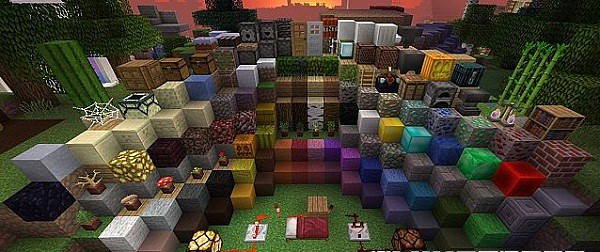The image depicts a vibrant, computer-generated landscape that resembles the pixelated style of Minecraft. The foreground features an array of colorful, textured blocks, forming a V shape that rises from the bottom corners to the center. These blocks display a vivid spectrum of colors, boasting shades of orange, red, pink, purple, blue, green, and yellow, reminiscent of a pride celebration. The blocks have various patterns on them, including brick, stone, slate, marble, stripes, and checks. Some blocks are adorned with small details like red and white mushrooms, green plants, a white spider web, and an hourglass. Additionally, lucky bamboo stalks are visible among the boxes. Behind this intricate construction lies a cityscape bathed in the warm hues of an orange sunset, with yellow tones illuminating the sky, adding depth and atmosphere to the scene.